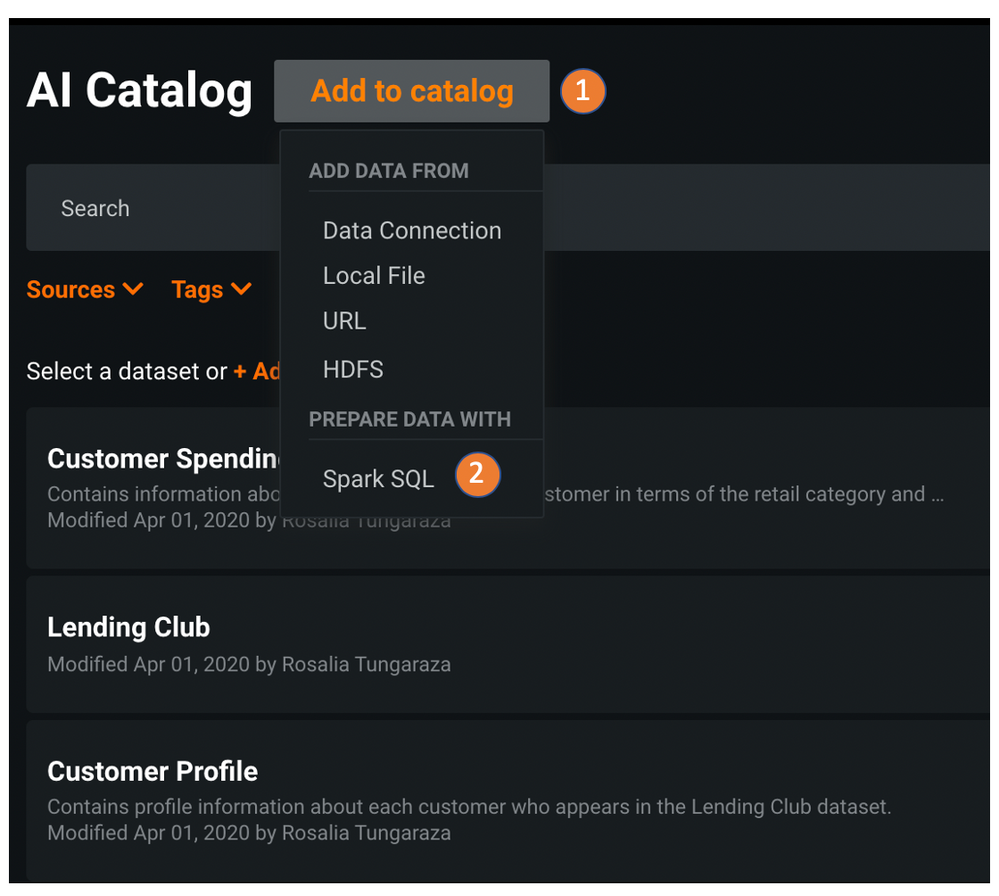The screenshot displays an interface with a black background. In the top left corner, white text reads "AI Catalog," and to its right, an orange, grayed-out button states "Add to Catalog." Below this is a menu item in gray text reading "Add Data From," listing options such as "Data Connection," "Local File," "URL," and "HDFS."

Further down, there's a section labeled "Prepare Data With" followed by "Spark SQL," accompanied by a small orange circular icon with a white "2" inside it. Adjacent to the "Add to Catalog" button, another orange circular icon displays the number "1" in white text.

Behind this main menu, a gray search bar labeled "Search" appears on the left. Below the search bar are two orange drop-down menus: one labeled "Sources" with a downward-pointing triangle, and another labeled "Tags" with the same triangle icon.

Beneath these menus, white text states "Select a Dataset or plus," followed by partially obscured text starting with "AD." Below this, another heading, partially visible, likely reads "Customer Spending." The menu covers part of this text, showing only "Customer" and an incomplete word. Further description suggests it contains information about customer behavior in the retail category but is truncated.

The next visible element is a card titled "Lending Club" in white text, with a gray subheading stating it was "Modified April 01, 2020 by Rosalia Tunggarasa." Below, another card labeled "Customer Profiles" describes its contents as "Contains Profile Information by Each Customer Who Appears in the Lending Club Dataset," and it was also modified on the same date by Rosalia Tunggarasa.